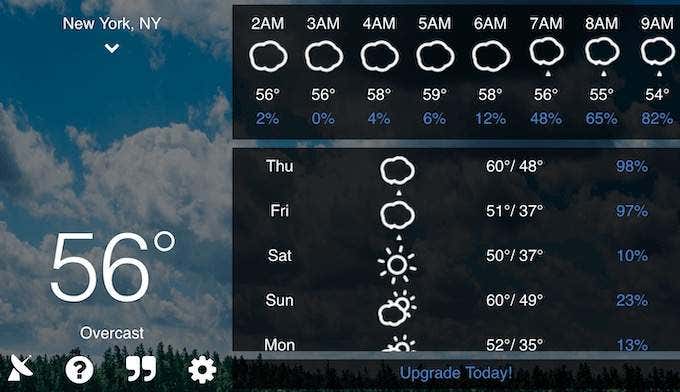A detailed and descriptive caption for the image could be:

"This is a cropped screenshot from a weather application, likely from a mobile device due to the prominence of the text size and absence of extensive user interface elements. At the top left, the location for the weather update is identified as New York, New York. Just beneath this, the current weather condition is stated as '56 degrees, overcast.'

The forecast for the early morning hours from 2 a.m. to 9 a.m. is detailed below, starting with a steady temperature of 56 degrees at both 2 a.m. and 3 a.m. The temperature then rises to 58 degrees at 4 a.m. and peaks at 59 degrees at 5 a.m. Following this, there is a gradual decrease: 58 degrees at 6 a.m., 56 degrees at 7 a.m., 55 degrees at 8 a.m., and finally 54 degrees at 9 a.m. The percentage shown alongside these times signifies the chance of rain, which starts at 2% at 2 a.m. and incrementally increases to 82% by 9 a.m.

Further down, the weather forecast for the coming days is displayed, starting with an expected 98% chance of rain on Thursday and 97% on Friday. The likelihood of rain then drops significantly over the weekend, with a 10% chance on Saturday, 23% on Sunday, and 13% on Monday.

The bottom left corner features a set of touch buttons depicted as icons: a satellite dish, a question mark within a circle, quotation marks, and a settings cogwheel. Additionally, there is an 'Upgrade Today' button, although it does not specify the feature to be upgraded.

The background of the image showcases a serene treeline set against a slightly cloudy yet bright sky, adding a picturesque touch to the functional weather display."